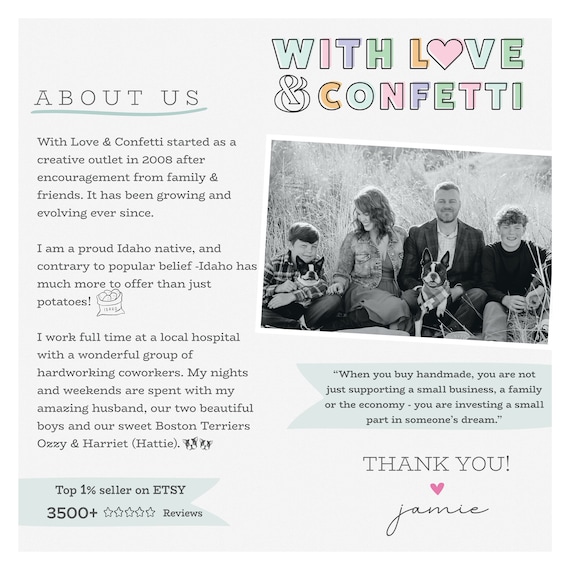This is an "About Me" design card for an Etsy shop called With Love & Confetti. At the top right in vibrant alternating colors of light blue, pink, purple, green, and orange, the card boldly declares "With Love & Confetti," with the "O" in "Love" shaped like a heart. On the left side, the heading "ABOUT US" is presented in all caps with a blue curved line beneath it. Below this, the narrative explains that With Love & Confetti began in 2008 as a creative outlet encouraged by family and friends, and has been thriving and evolving ever since. 

The heartfelt description details that the shop owner is a proud Idaho native who takes pride in her state's offerings beyond just potatoes. She works full-time at a local hospital and cherishes her evenings and weekends with her family—her supportive husband, her two wonderful boys, and their beloved Boston Terriers, Ozzie and Harriet (also known as Hattie). 

An accompanying black-and-white photograph showcases the family: a smiling woman looking fondly at her younger son holding one of the dogs, the husband smiling at the camera, and an older son who appears to be about 14, with another dog in front of them. 

Decorative elements include a medium blue ribbon stamp on the bottom left, indicating the shop's recognition as a "Top 1% Seller on Etsy" with over 3,500 five-star reviews. Adjacent to the photograph, a drawn image of a sack of potatoes and two Boston Terrier faces add a personal touch. Below the family photo on a light blue background is an uplifting quote: "When you buy handmade, you are not just supporting a small business, a family, or the economy. You are investing a small part in someone's dream." The card ends with a heartfelt "Thank You" and a pink heart, signed in cursive by Jamie.